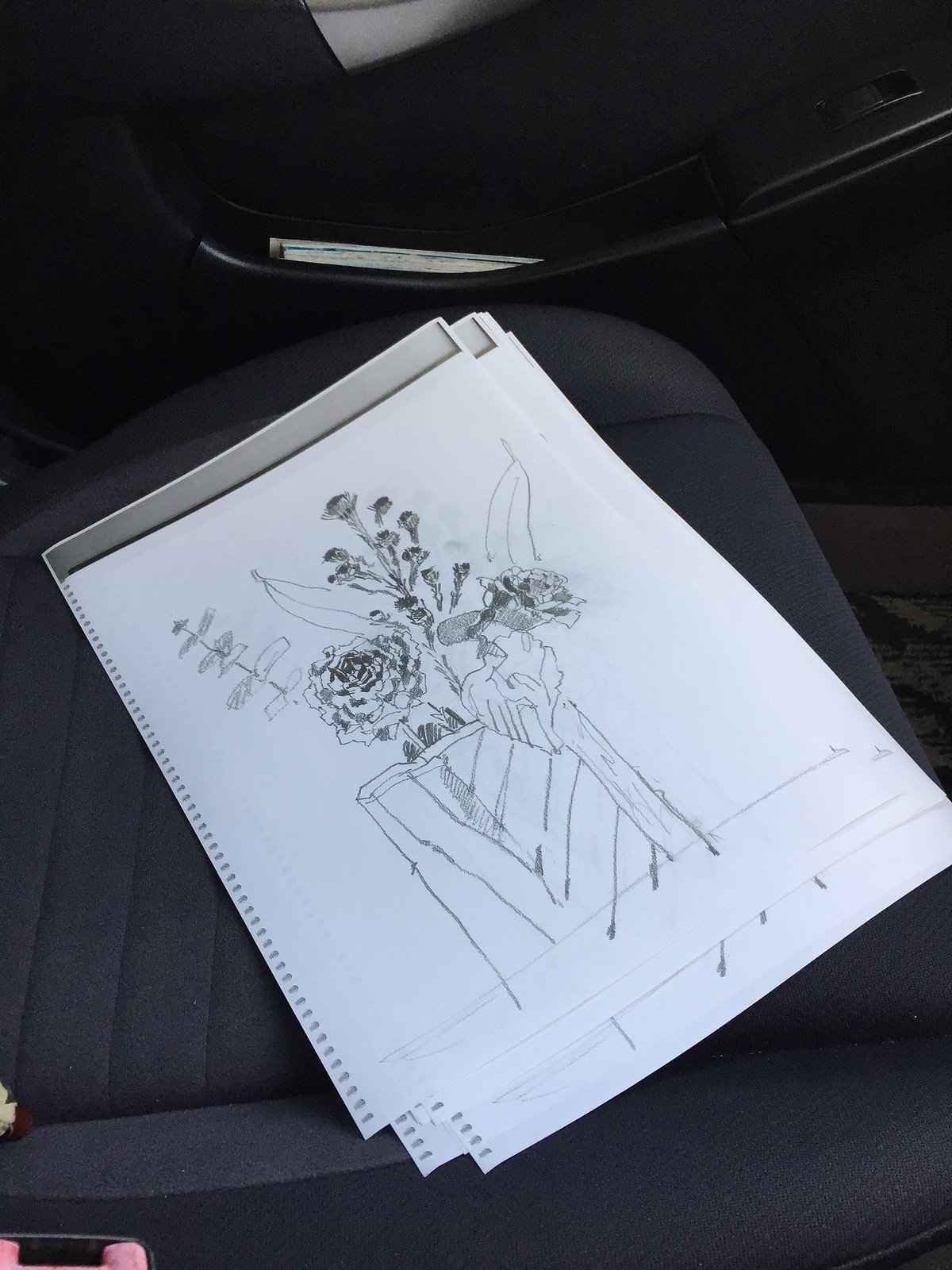The image showcases the front passenger seat of a car with a dark gray interior, including a visible seat belt receiver and a car door featuring a side pocket filled with maps. Lying on the seat are several rectangular sheets of drawing paper, previously part of a spiral-bound sketchbook as indicated by the perforated holes along their left edges. The focus is a detailed pencil drawing on top, depicting a podium-like base or possibly a plastic bag, from which a variety of flowers and leaves of different shapes and sizes emerge. Among these, a rose is prominently featured, alongside other large flowers and leaves, rendered in various shades of gray to convey depth. The scene is enriched by elements such as a black-and-pink object on the bottom left of the image and some silver accents visible on the car door above the seat.